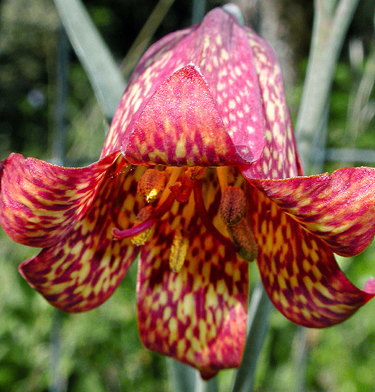This professionally shot full-color outdoor photograph, taken during the daytime, centers on a unique, downward-facing flower with very large, open petals. The square image captures the flower in intricate detail, showcasing its predominantly purple petals accented with vibrant yellow splashes. The flower is fully open, revealing its pollen-laden interior, but no bees or insects are present. Set against a softly blurred background of green foliage and plant stalks, the photo emphasizes the artistic beauty and natural environment of the flower.